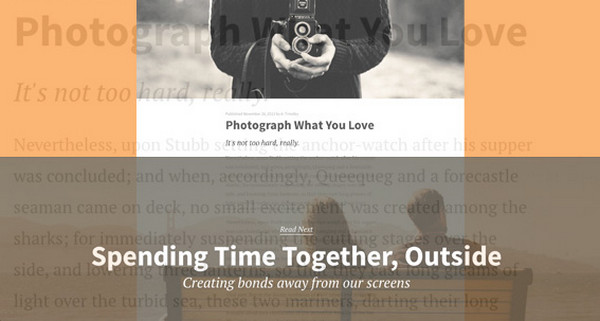This image displays a website with various elements designed to encourage and illustrate the concept of capturing meaningful moments through photography. Dominating the visual presentation is a prominent orange box that frames a black-and-white photograph. The photograph features a person dressed in a black sweater, clutching an old-fashioned, handheld camera and adjusting its zoom. Interestingly, only the person's torso is visible, leaving their head and the rest of their body out of the frame. Below this photograph, a white box clearly displays the text: "Photograph what you love. It's not too hard really."

Underneath the white box, a grayish-brown shaded section occupies the lower part of the image. This part features a secondary photograph showing a man and a woman seated on a bench. The man is gazing to the right, while the woman looks straight ahead. This image is captioned with the phrase: "Spending time together, outside," followed by a smaller white text underneath that reads: "Creating bonds away from our screens," which adds a touching and meaningful layer to the content.

Despite the detailed and expressive content, the image and the website lack any contact information, such as a phone number or web address, which is somewhat unexpected. Additionally, the background contains a paragraph that elaborates on the theme of capturing moments, adding depth and context to the visual and textual elements presented.